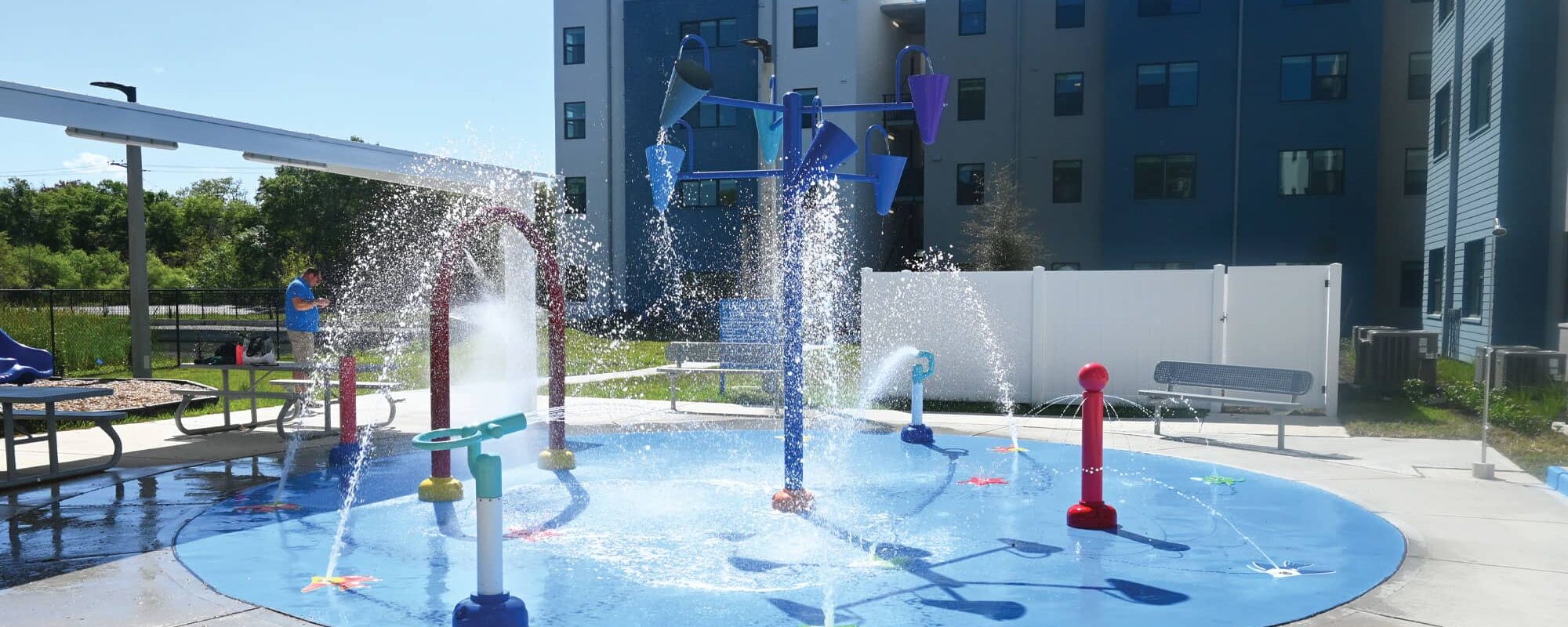The image captures a vibrant blue splash pad centered around a blue-colored pole, with streams of white water spraying onto the pad. The water sprays create dynamic white streaks against the blue surface, adding a lively feel to the scene. In the background, a series of buildings in various shades of navy blue and gray provide a striking contrast to the splash pad. These buildings are adorned with rectangular windows, contributing to the urban atmosphere. A distinctive red cylinder, embedded in the ground near the splash pad, adds a pop of color to the overall composition.